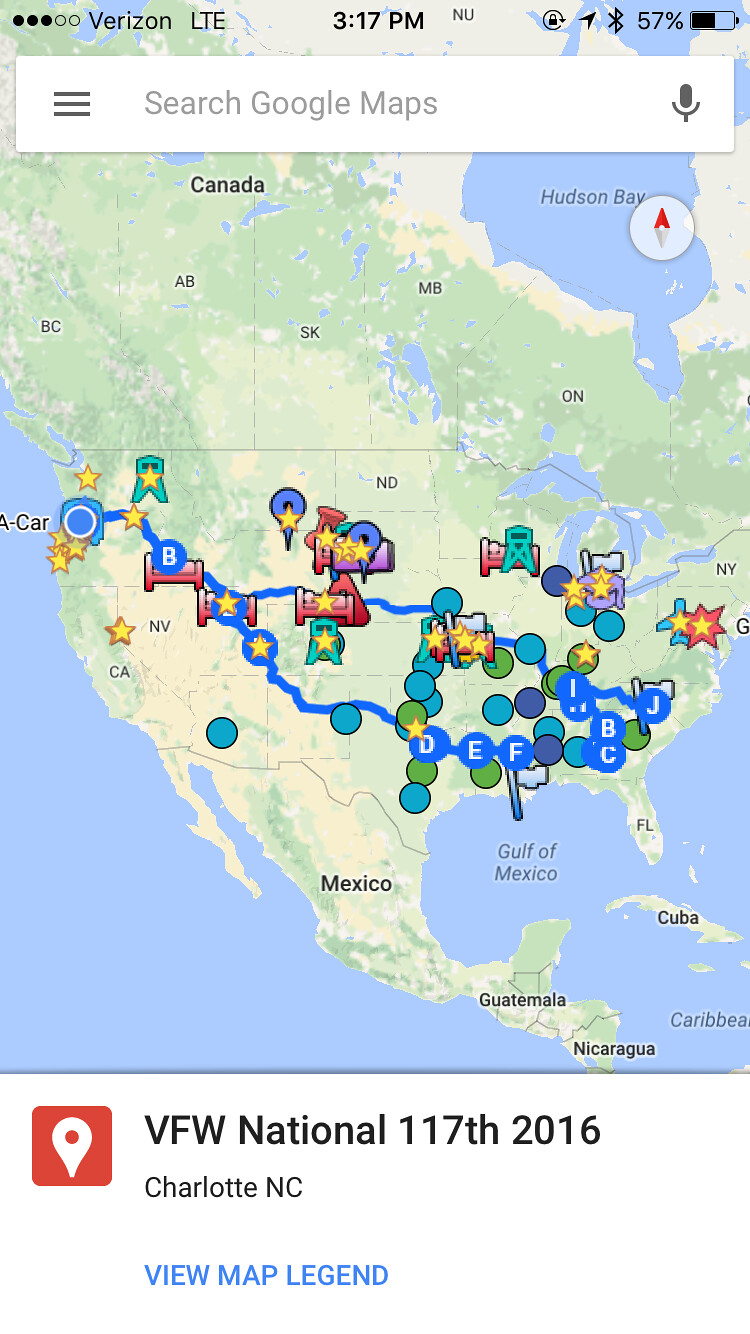This image is a detailed screenshot from a smartphone displaying Google Maps. At the top of the screen, indicators show it is 3:17 PM with Verizon LTE connectivity and a 57% battery level. The Google Maps search bar appears below, complete with a hamburger menu icon and a microphone symbol.

The main image showcases North America, covering Canada, the U.S., Mexico, and several Central American countries, such as Guatemala, Nicaragua, and Cuba. Prominently featured is a large blue loop traversing the United States, suggesting a route with various stops. These stops are marked by a variety of symbols, including circles, beds, stars, and possibly water towers, each potentially indicating specific locations or amenities. Along the blue route, white letters—J, B, C, F, D, I, E, B—appear at different points, possibly denoting points of interest or directions.

Towards the bottom of the image, a label reads "VFW National 117th, 1-17-2016, Charlotte, NC," with a prompt in blue text to view the map legend, enhancing the understanding of the depicted path and symbols.